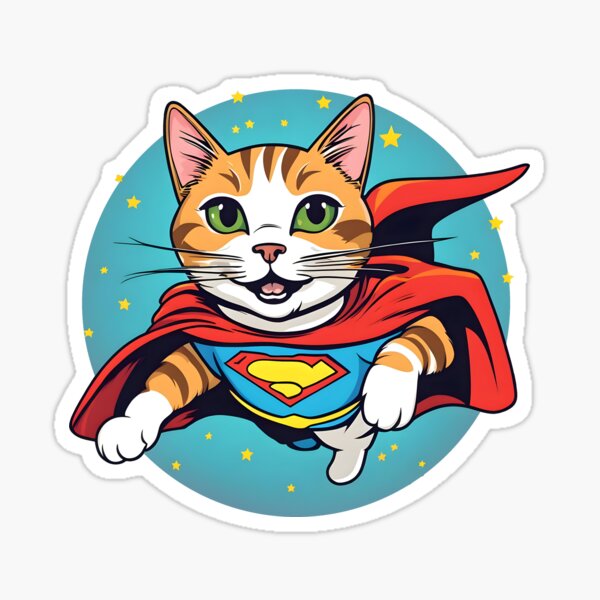The cartoon image features a cheerful, flying tabby cat dressed in a Superman-style outfit. The cat, with a white face and signature pink nose, sports prominent black whiskers and lively green eyes with black pupils. Its outfit includes a blue top adorned with a red diamond logo, a yellow belt, and white boots. A vibrant red cape flutters dramatically behind it. The cat appears to be zooming through an airy background of baby blue, dotted with scattered yellow five-pointed stars. Surrounding this lively scene is a lilac-hued border, adding an extra layer of whimsy. The cat's head is framed by brown and orange bangs, and its expression radiates joy and excitement as it appears to be soaring through the sky.